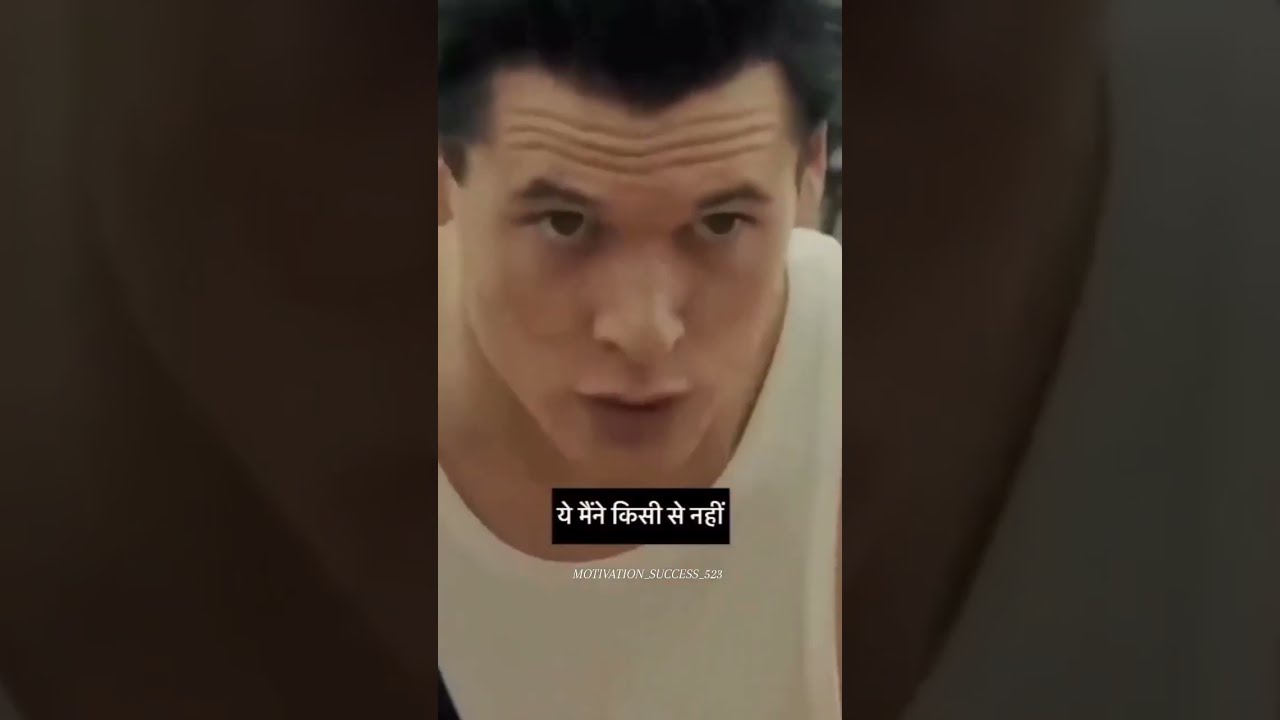The image is a wide, rectangular screenshot from a film or video clip featuring a white male with black hair, slightly balding, and light skin. He is wearing a white t-shirt and his face shows an intense focus, with three thick creases on his forehead and his eyebrows raised. His mouth is slightly open, but his teeth are not visible. The man has brown eyes and his head is slightly leaning forward as he looks off towards the right-hand side of the image. The central part of the screenshot displays his face prominently, while darker, zoomed-in sections of his neck and chin are shown on either side of the main image, creating a composite effect.

Beneath the man's chin in the screenshot, there is a black rectangle with foreign lettering, possibly Asian or Taiwanese. Below this black bar, in white font, it reads "Motivation Success." Additionally, smaller text, "motivation_success_523," appears at the bottom of the image. The overall composition suggests that this could be a cell phone or mobile phone screenshot of a video, with all elements oriented upright.